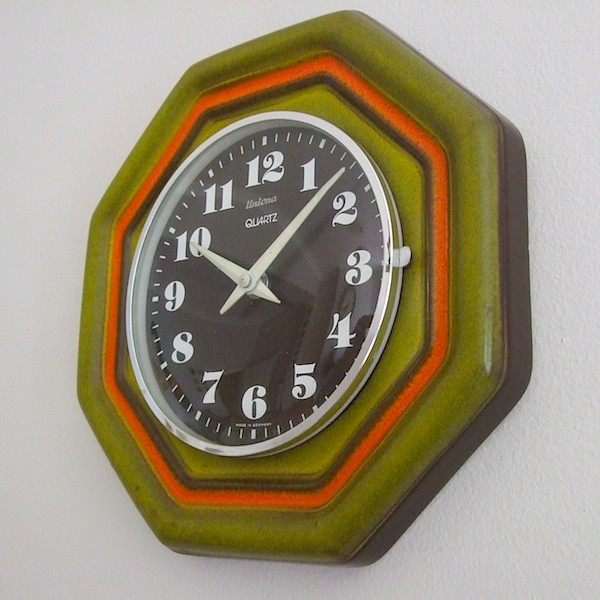The photograph features a retro-styled analog clock mounted on a white wall, slightly angled in the frame. The clock has a striking design with multiple octagonal layers: the outermost layer is olive green, followed by an orange octagon, and then another olive green octagon, all forming concentric shapes. The clock face itself is circular with a silver edge and features a black background with white numerals and hands, indicating the time as approximately 7 minutes past 10 o'clock. The word "quartz" is prominently displayed at the center. Notably, there is a small tab on the side of the clock face, suggesting ease of battery replacement. The overall color palette includes army green, olive green, orange, and hints of brown on the outer edges, giving the clock a distinctive vintage appearance.